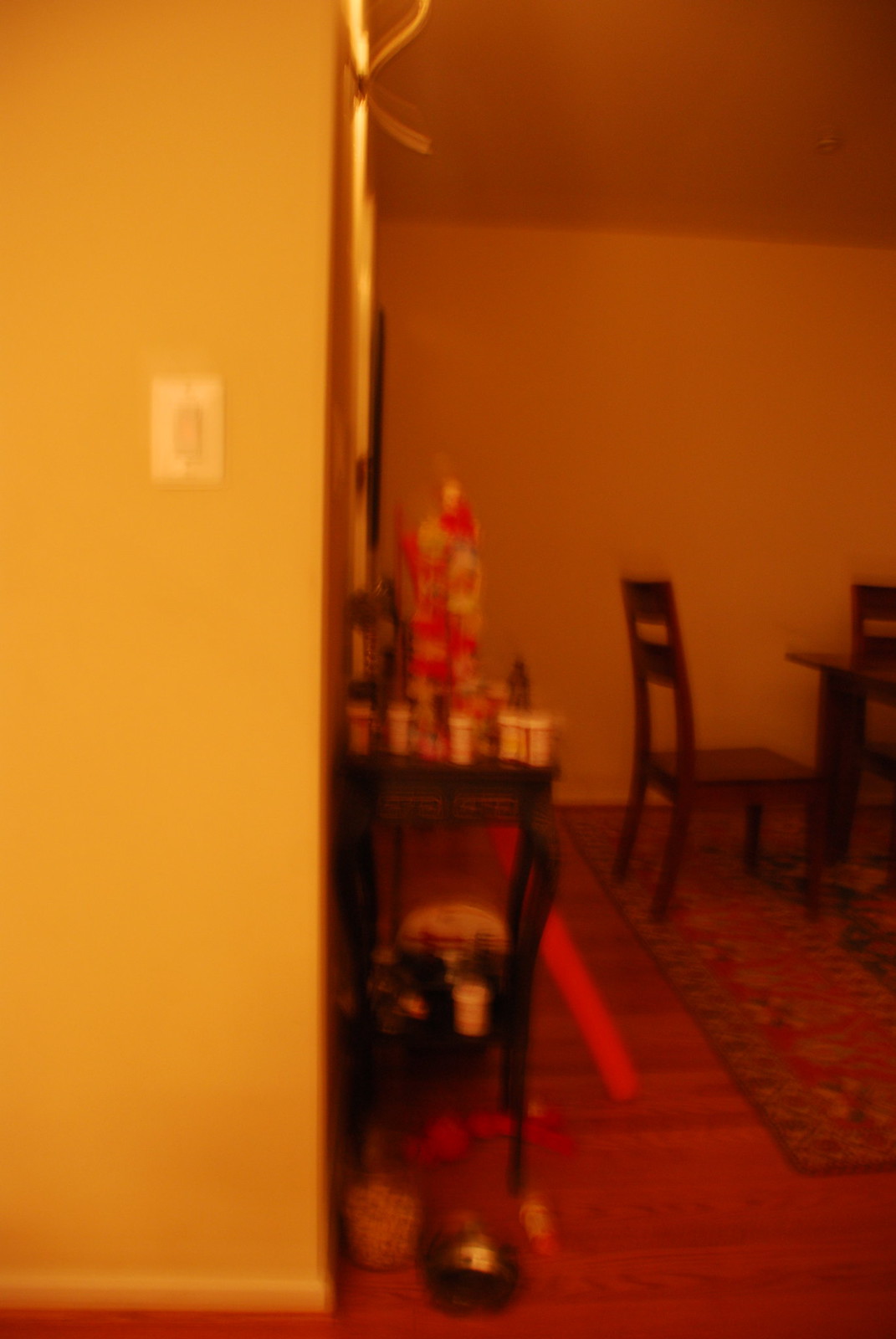The image depicts a slightly blurry and low-quality photograph of an interior space, primarily focused on a living room section that is partially cut off on the right. On the left side, the image captures a white wall that serves as a partition between the dining room and another adjacent room. This wall occupies approximately 45% of the left side of the frame and features an electrical outlet. At the bottom of the wall, there is visible finished wood flooring that extends into the adjoining room. Emerging from the right-center of the image is a wooden dining table, with a single chair that appears to be pulled away from the table, positioned prominently in the center of the shot.